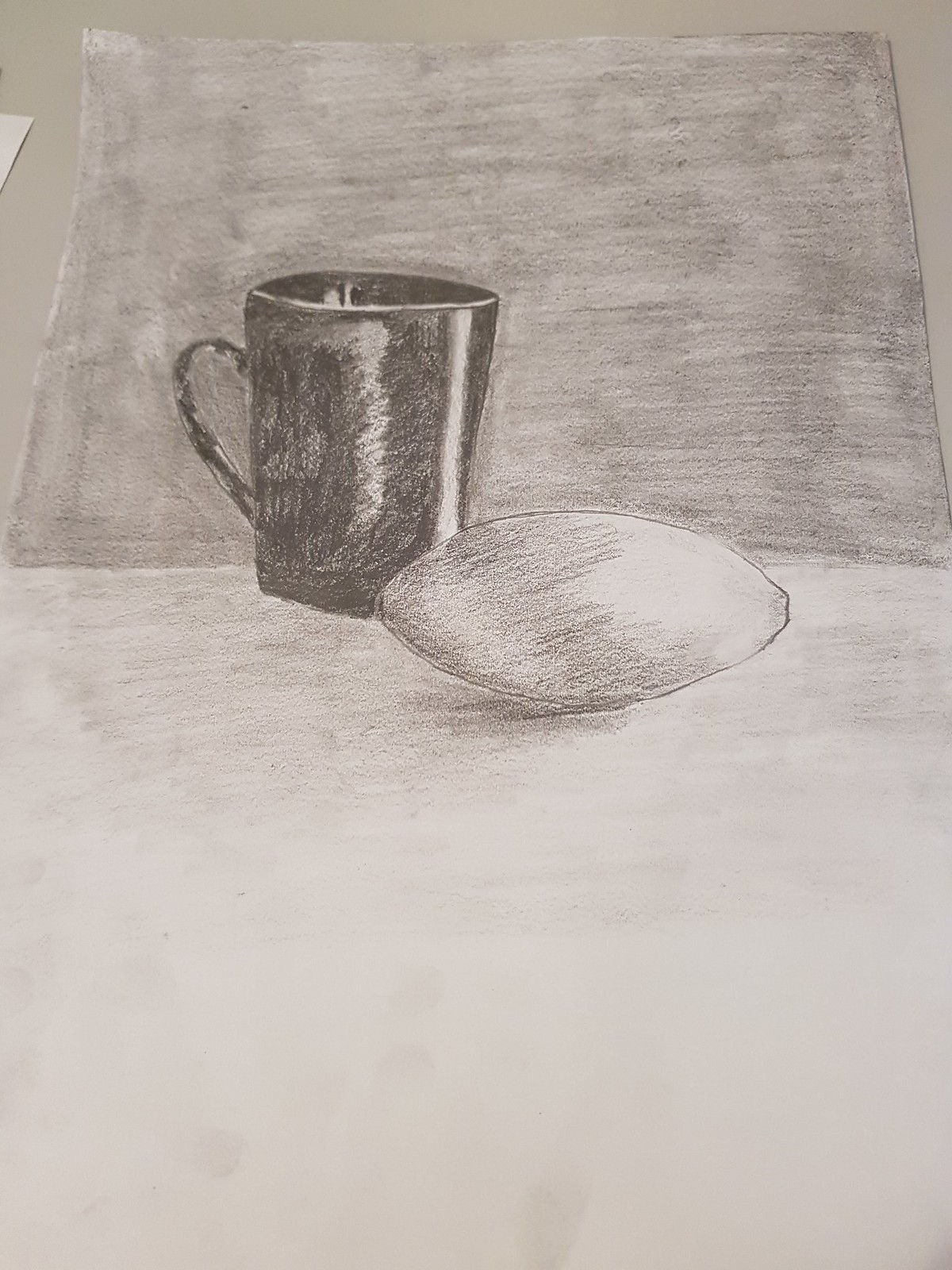In this detailed black-and-white pencil drawing, a meticulously shaded black coffee mug with a rounded handle sits prominently on a white surface, slightly left of center. The mug, which reflects light to reveal a glossy sheen, allows a faint glimpse inside. Placed slightly to the mug's right and lower, an oblong object resembling a lemon rests on the surface. The lemon, with its smooth, elongated form, contrasts against the mug’s dark hue.

The background comprises a hemmed, plain tea towel draped across the top half of the image, its beige tint hinted subtly through light pencil shadings. The towel does not extend to touch the edges of the frame, creating a sense of incompleteness. The surface below is mostly white, with sparse pencil marks adding texture. The overall composition, rich in grayscale, captures a quiet still life, reflecting careful attention to light, shadow, and texture.